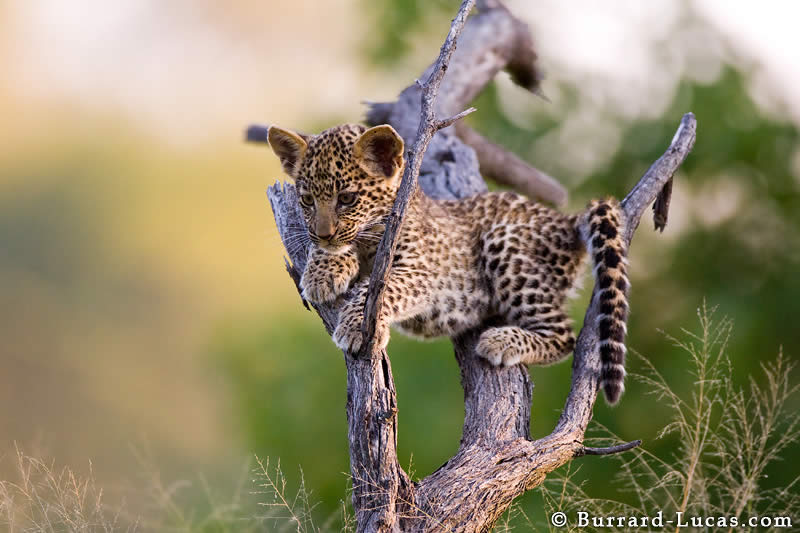The image captures a very cute and tiny leopard cub, possibly a baby cheetah but more likely a leopard, with a golden coat adorned with numerous black spots. The cub is perched high on a bare, dead tree branch, seemingly away from the ground. It is positioned with its paws on one branch, its body draped over another, and its tail leaning on a third branch. The cub appears to be gazing intently downwards, perhaps at something in the bottom left corner of the camera frame. Its ears are perked up, and it looks relaxed with its head resting on its paw. In the background, there are blurry green and yellow hues suggestive of trees, alongside skies that transition from white at the top to an orange-yellow towards the bottom, indicating a sunset. The photo also contains some text at the bottom right corner that reads "copyright burrard-lucas.com." The overall lighting suggests it is a nicely lit day, casting a natural spotlight on the adorable cub.